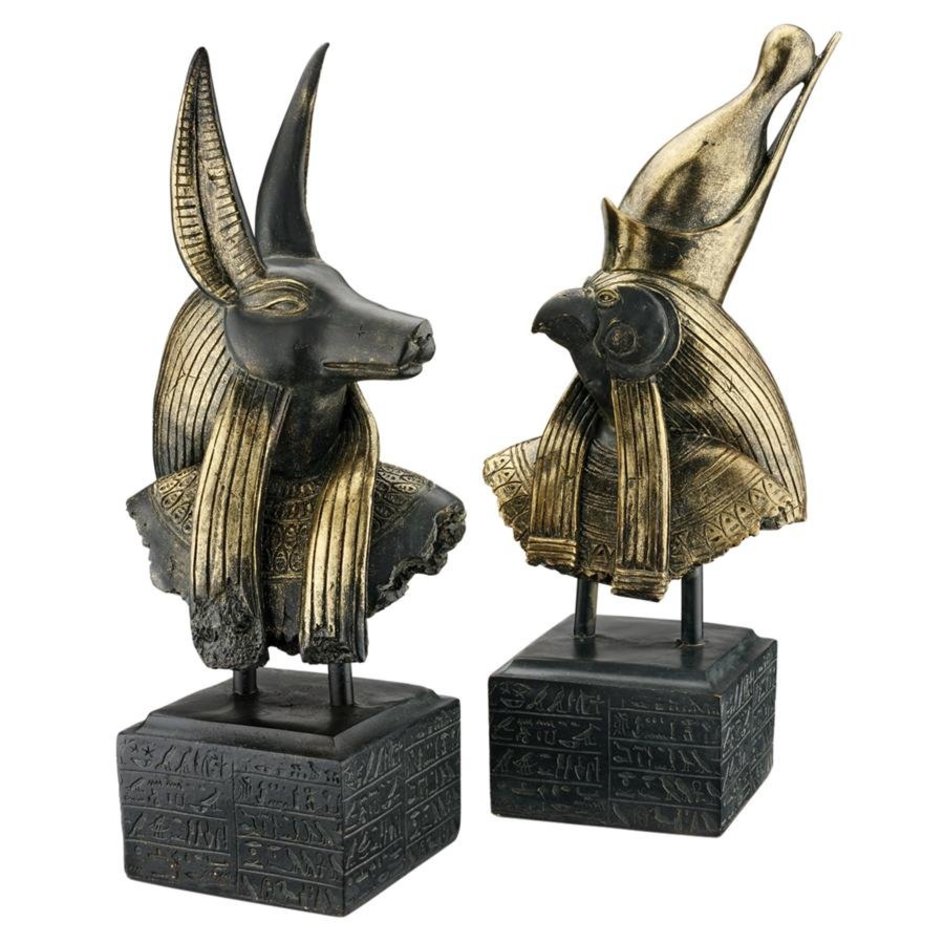This photograph showcases two intricate mini sculptures with distinct Egyptian features, positioned against a seamless white background. Each sculpture is perched on identical black square bases adorned with ancient Egyptian hieroglyphics. The sculptures, primarily black with gold and bronze accents, are mounted on dual black rods extending from the bases. 

The sculpture on the left represents a deity with the head of a jackal, characterized by its tall, pointed ears and elongated snout. It is draped in a cloak-like garment, with additional ornamental elements flowing behind its head. A wide, ornate collar or chest piece featuring hieroglyphics further adorns the figure, adding to its regal appearance.

The sculpture on the right depicts another deity, identified by its bird-like head and pronounced beak. This figure sports a large headpiece with a wave-like design extending back and down, embellished similarly to the jackal head. It also wears a striking collar decorated with hieroglyphics, enhancing its majestic look. Both sculptures face each other, emphasizing their divine presence and symbolic significance within ancient Egyptian culture.